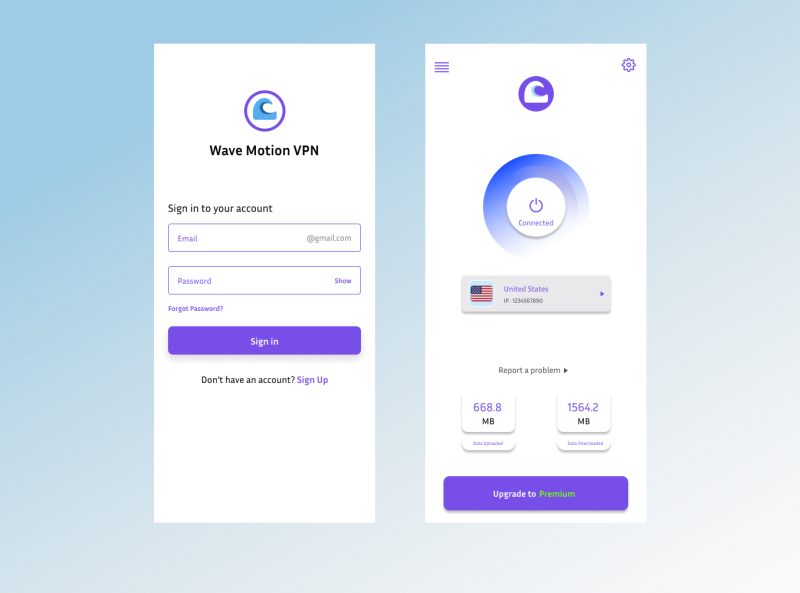### Descriptive Caption

Two phone screenshots showcasing the user interface of the Wave Motion VPN app:

**Left Screenshot:**
- The interface displays the login screen for Wave Motion VPN.
- At the top is a small purple circle featuring a water wave icon.
- Below are fields for email and password, each outlined in purple rectangles, with a "show password" button situated to the right of the password field.
- Underneath these fields is a "Forgot Password?" link.
- Further down is a purple button with white text labeled "Sign In."
- Beneath this, there is an option to "Sign Up" for new users, written in purple text.

**Right Screenshot:**
- The second image displays the main control screen after logging in.
- A contact menu is located on the bottom left and a settings menu in the upper right, both in purple.
- The top also features the same purple logo seen in the login screen.
- A power button indicating "Connected" is outlined in blue.
- Shows connected to a mock IP address: 1234567890, indicating a United States server.
- Contains a "Report a Problem" option for user feedback.
- Displays data metrics: "6668.8 MB" of data used and "1554.2 MB" of data remaining, with the MB units in black.
- At the bottom, there is an "Upgrade to Premium" button, with "Upgrade to" in white and "Premium" in green text on a purple background.

The background for both screenshots is sky blue, providing a uniform and clean visual context for the app’s features.